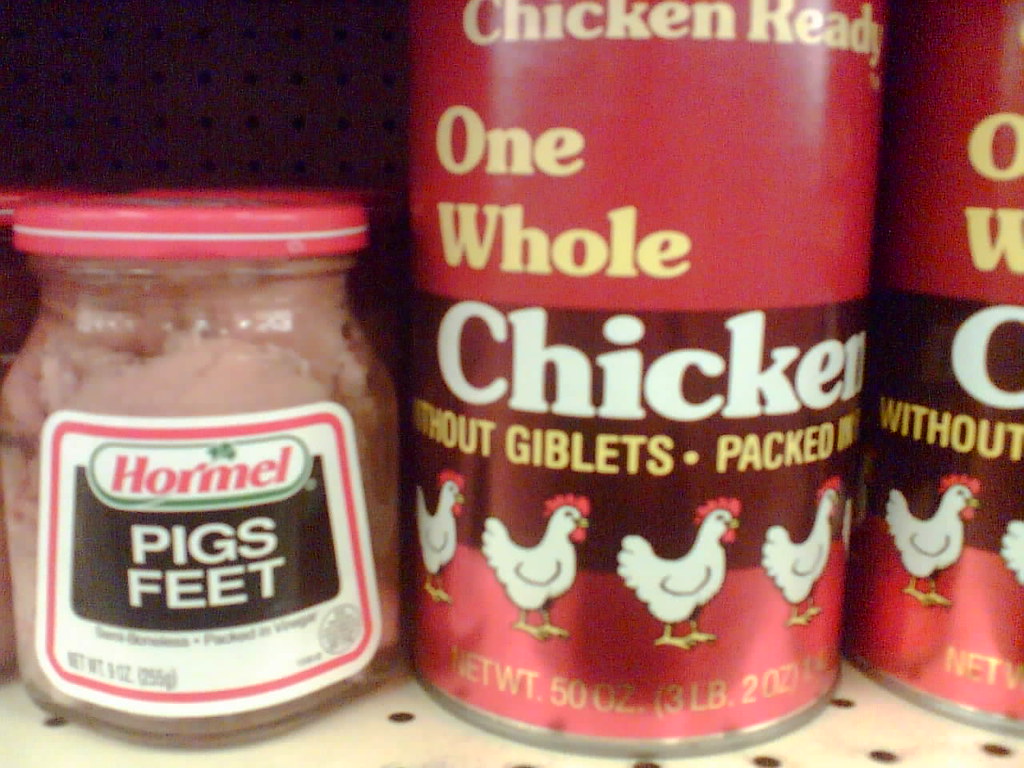The image displays a zoomed-in view of a grocery store shelf with a white surface having small holes and a dark brown background. On the left, there is a glass jar labeled "Hormel" containing pig's feet. The jar is transparent with a light red cap that has a white circle through it. The label features the word "Hormel" in red letters surrounded by green and below it, in white letters on a brown background, it says "Pig's Feet." Next to this jar are two identical tall red cans labeled "Chicken Ready." These cans feature the text "One whole chicken without giblets packed" in yellow letters against the red background, with "chicken" written in large white letters on a brown section. The net weight is marked as 50 ounces or 3 pounds and 2 ounces. The cans also display small white chickens with red combs. The items are positioned on a typical grocery store shelf, suggesting they are affordable food options.